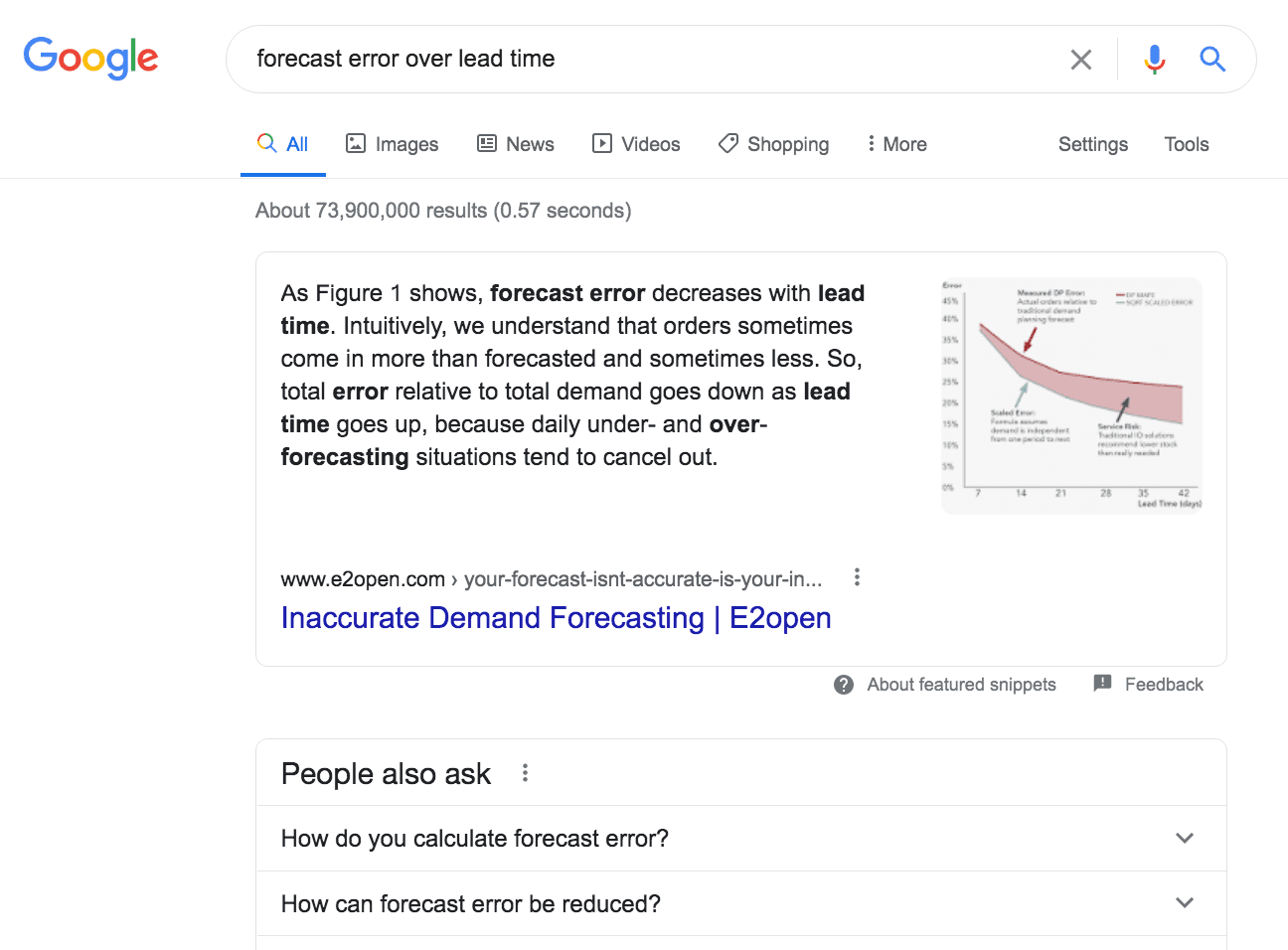This detailed caption for an image of a Google search page has been provided below:

---

This is a comprehensive screenshot of a Google search results page. At the top left corner, the Google logo is displayed in its distinctive colors: blue, red, yellow, blue, green, and red. The search query entered in the prominently centered search bar reads "forecast error over lead time". The selected search category is "All," with other options available such as Images, News, Videos, Shopping, More, Settings, and Tools. 

The results summary beneath the search bar indicates approximately 73,900,000 results were found in 0.57 seconds. A highlighted snippet from e2open.com is featured prominently, beginning with the statement, "As figure one shows, forecast error decreases with lead time. Intuitively, we understand that orders sometimes come in more than forecasted and sometimes less. So total error relative to total demand goes down as lead time goes up because daily under and over forecasting situations tend to cancel out." Adjacent to this description is a graphical representation.

Below this section, the link to the source is listed as www.e2open.com, along with a truncated page title, "Arrow, your forecast isn't accurate is your in..." followed by "Inaccurate demand forecasting / e2open". The image also contains options for "About featured snippets" and "Feedback."

In the "People also ask" section, users are prompted with questions such as "How do you calculate forecast error?" and "How can forecast error be reduced?" The image does not feature any people or animals.